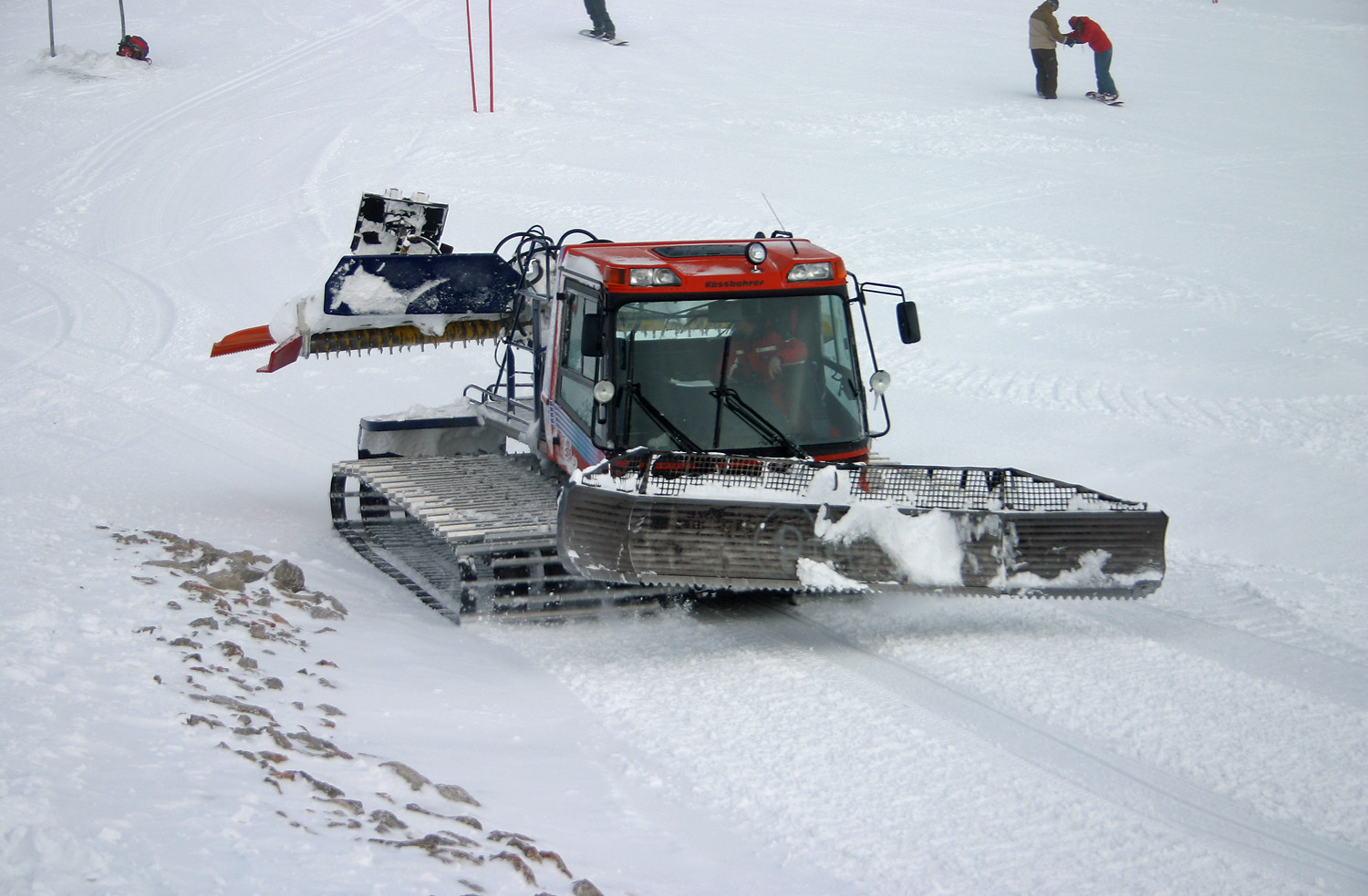In this detailed image of a snowy slope, the scene unfolds on a cold winter day with a blanket of white snow covering most of the landscape, except for a small rocky patch in the lower left corner. A vibrant red snow groomer with a large blade at the front and a scraper at the back dominates the foreground. The machine, likely used for compacting and smoothing the snow on the ski slope, features a spacious glass-enclosed cab. The operator inside, wearing a red and white snowsuit, focuses intently on his task.

A little further up the hill, three people can be seen. One snowboarder is being helped by another person standing behind them, indicating a moment of assistance or instruction. The person giving support wears a red jacket, matching the dominant color theme of the machinery and operator's outfit. The third individual, only partially visible, showcases their legs and snowboard, suggesting they are either preparing to descend or have just completed their run. Additionally, a series of orange poles stick up from the snow, likely marking the ski trail boundaries. The overall scene captures a bustling and functional slice of life on a snowy ski slope infused with vibrant red accents amidst the predominant white landscape.